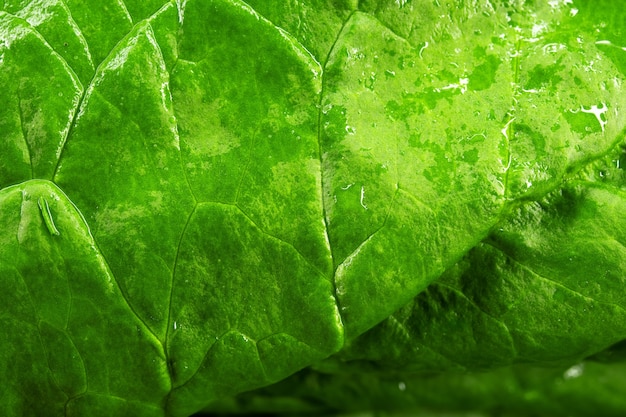This image captures an extreme close-up of a vibrant, green leaf, showcasing intricate details and varying shades. The photograph focuses on the leaf's veins and the fine, porous texture. The hues range from light to dark green, adding depth and complexity to the overall image. In the center, a small separation between sections of the leaf is visible, highlighting the plant’s natural structure. Moisture is evident, particularly in the upper corner, where the leaf glistens with wetness. The bottom right of the image is slightly out of focus, which may be due to water reflection or simply an inherent blur. Additionally, the upper right displays subtle white markings, perhaps suggesting the leaf has been scratched. The leaf might be from a tree, flower, or even something edible like lettuce or spinach, but its specific type remains indistinguishable due to the close-up nature of the photograph.